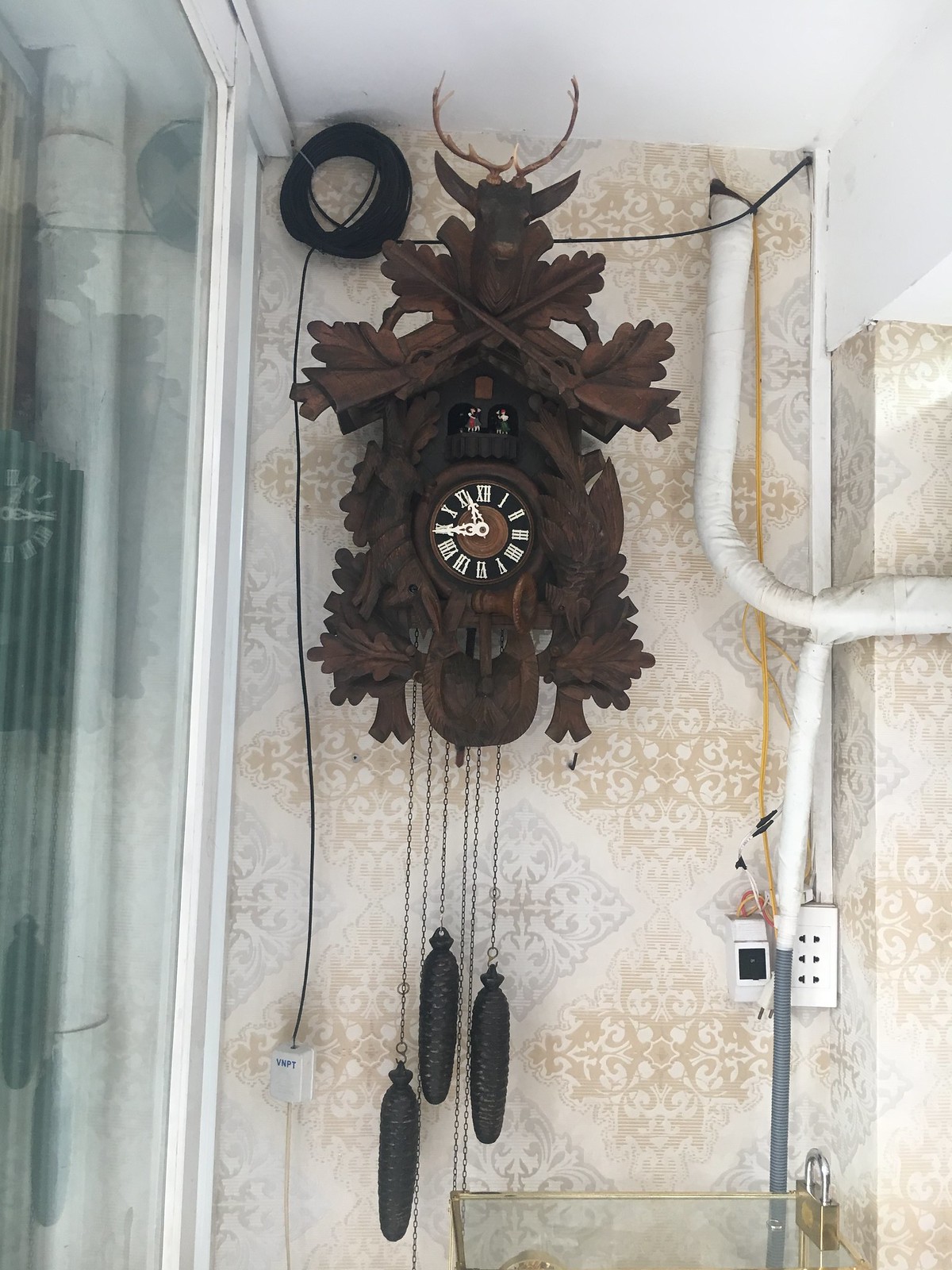This photograph captures the interior of a room featuring an intricately detailed cuckoo clock mounted on a wallpapered wall with a light diamond pattern. The rich, dark-brown wooden clock appears to be hand-carved, showcasing a nature and hunting theme. At the top of the clock, a deer with light brown antlers is mounted, and underneath it, two rifles are crossed above an axe, all nestled within ornate floral and leafy designs. Below these figures is a platform where two small figurines, either a boy or a girl, emerge to perform at various times. The clock face is adorned with bright white Roman numerals and clock hands, and underneath, three intricately designed pine cone weights hang from chains, indicating the traditional mechanics of the cuckoo clock.

The room also includes a glass door on the left side and an unusually prominent VNPT-labeled box with a bundle of black cables protruding from another room, some of which are tied up in the upper left corner. There is some electrical conduit visible to the right of the clock. The combination of an ornate antique clock and modern wiring against the backdrop of the light diamond-patterned wallpaper creates a striking contrast in this indoor setting. The time displayed on the clock is approximately 11:45.